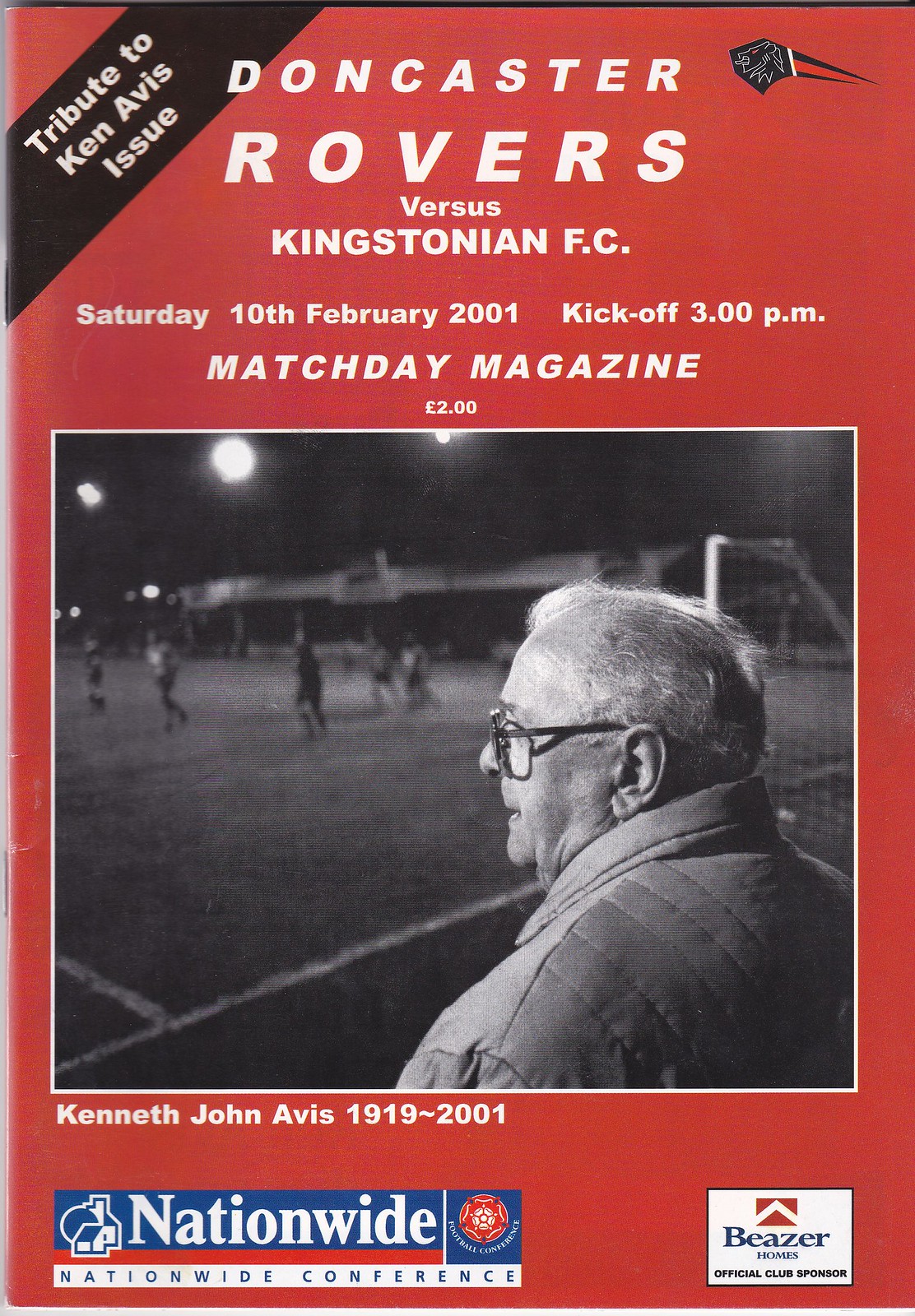The cover of this rectangular sports program features a predominantly red background with white print. Dominating the center is a black-and-white photograph of an elderly man wearing glasses and a coat, who is gazing onto a soccer field lit under a dark sky, with scattered players and a goal post visible to his right. The title at the top reads "Doncaster Rovers versus Kingstonian FC, Saturday, 10th February 2001, kickoff 3 p.m., Match Day Magazine" priced at £2. A black banner in the top left corner annotates this as a "tribute to Ken Avis issue." Below the photograph, his life span, "Kenneth John Avis, 1911-2001," is honored. The bottom of the cover highlights sponsors including the Nationwide Conference and Beezer Homes.